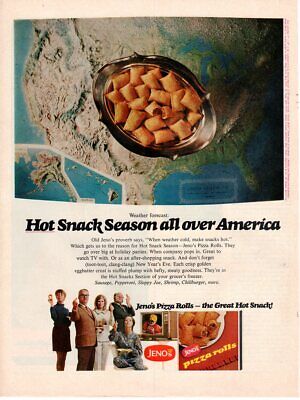This vintage magazine advertisement for Gino's Pizza Rolls, likely from the late 60s or early 70s, prominently features the bold headline "Hot Snack Season All Over America." The top half of the vertical ad showcases a silver bowl brimming with pizza rolls, one of which is cut open to reveal the cheesy, saucy filling. This bowl is intriguingly placed atop a detailed map of the United States, emphasizing the snack's nationwide appeal. 

Below this, at the base of the ad, a group of five individuals — comprising men, women, and a soldier — hold pizza rolls and gaze towards the camera, suggesting widespread enjoyment. To their right, a red box marked "Gino's Pizza Rolls" displays the brand's name and product description, with adjacent text that reads, "The Great Hot Snack." The predominant colors throughout the ad include blue, tan, green, red, black, and white, enhancing its retro 60s vibe. Additionally, there appears to be a small TV screen, further reinforcing the period's aesthetic.